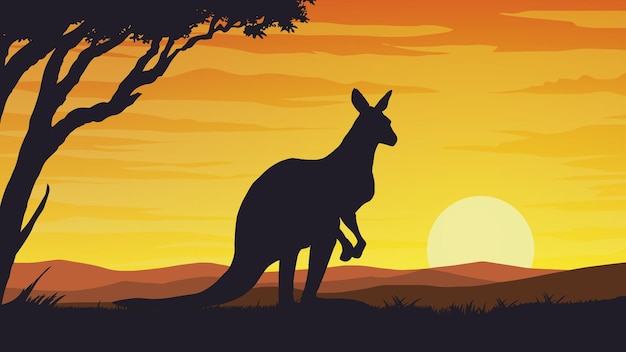The image depicts a high-quality, cartoonish illustration of a kangaroo standing in the center of a grassland at sunset. The silhouetted kangaroo, entirely in black, faces right with its short front legs lifted off the ground and its tail resting on the grass. The sun, a light yellow orb, is partially set on the right side of the image, casting a warm golden hue across the sky with streaks of orange clouds. To the left, a black silhouette of a tree with visible leaves extends from the edge of the horizontal-rectangular frame. The background features a brown mountain under the vibrant sunset. The scene, though dark in parts due to the silhouettes, is vividly brought to life with the contrasting warm colors of the sky, reminiscent of a high-quality animation, potentially from a Disney movie.